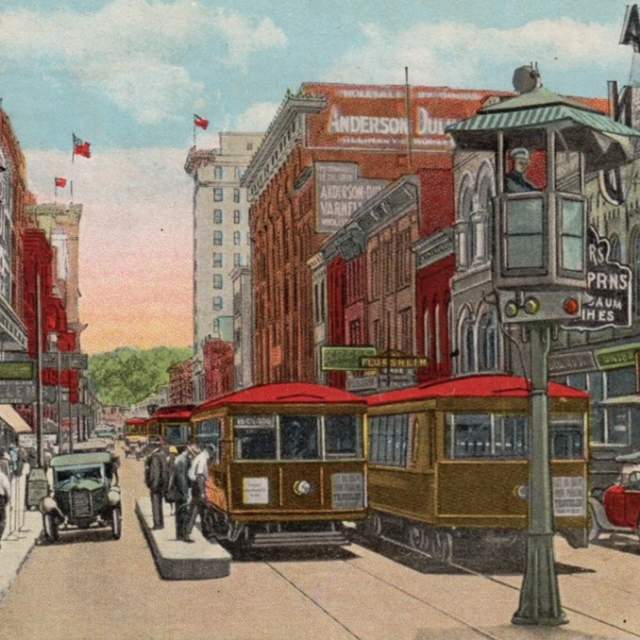This detailed colored sketch depicts a bustling small American town from the early 20th century, possibly the 1920s, based on the presence of vintage Ford model cars and red trolleys. The street scene captures a typical busy weekday, featuring several individuals waiting to board the streetcars. Prominently displayed is a man inside a control booth, likely managing the streetcar system. The architecture consists of brick office buildings in hues of white, red, pink, and orange, with signage such as "Flersheim" visible, though other texts are indistinct. Flags adorn some buildings, suggesting governmental significance. Background elements include a row of trees, suggesting either a park or the town's borders, while the sky transitions from a reddish-pink to blue, dotted with dispersed white clouds.